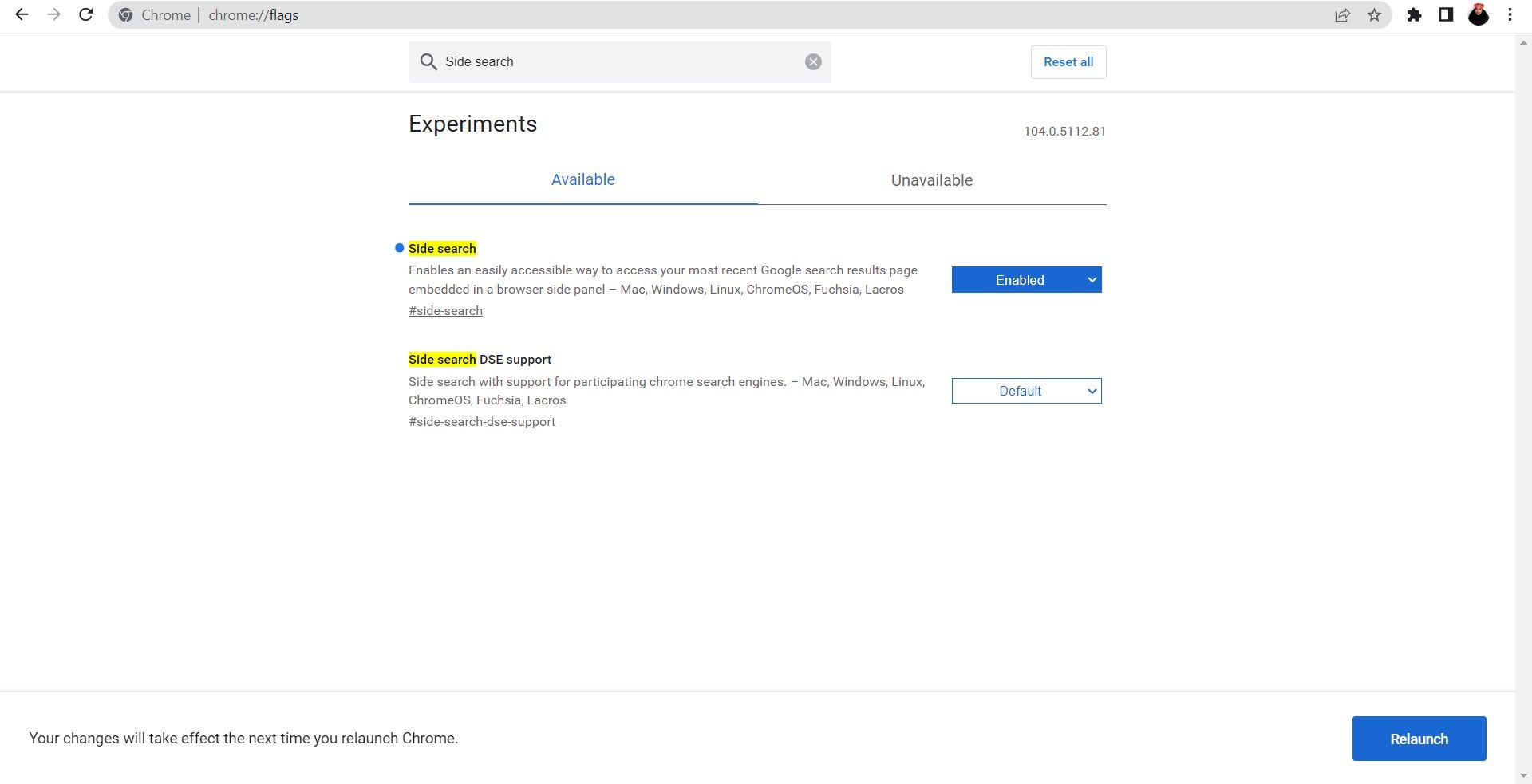Screenshot Description:

The screenshot displays a web page opened in the Chrome browser, featuring a sleek, Apple-like design with a white search bar at the top. Directly below the search bar, there's a settings menu designated for Chrome experiments. The menu is divided into two tabs: "Available" and "Unavailable," with the "Available" tab currently in focus.

Within the "Available" tab, although the text is largely illegible due to small font size and blurriness, the main header of the section is distinctly highlighted in yellow. To the right of this header is a blue "Enable" button that features a dropdown menu.

Further down, another section similarly highlighted in yellow appears with a button labeled "Default" beside it, which is white. At the bottom of the page, there's a notice stating, "Your changes will take effect the next time you relaunch Chrome," accompanied by a blue "Relaunch" button on the right side.